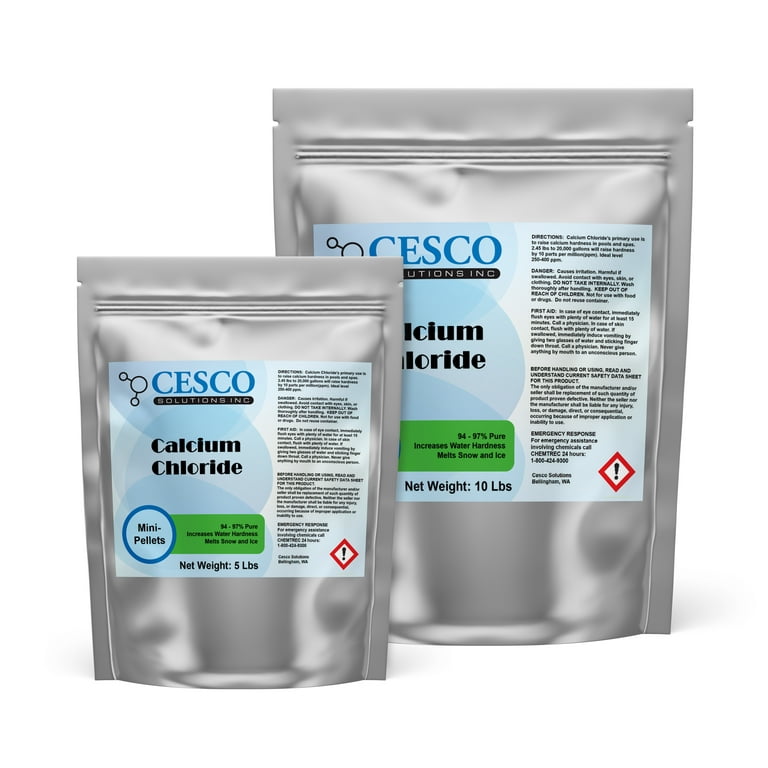This product photo features two silver, resealable plastic pouches of differing sizes positioned side by side. The smaller pouch, which weighs 5 pounds, is on the left and slightly overlaps the larger 10-pound pouch on the right, emphasizing its comparatively smaller size. Both pouches contain calcium chloride, marketed by CESCO Solutions Inc., with "CESCO" inscribed at the top of the label along with a logo resembling a water molecule. 

The label includes various details: beneath the brand name, the primary content "calcium chloride" is prominently displayed. Below that, there is a small circle featuring black text and a green box with additional writing. There are also four to five paragraphs of small black text to the right, detailing usage warnings and guidelines, though the text size makes it difficult to read. A distinguishing feature at the bottom right of the label is a red triangle with an exclamation mark inside, likely indicating a warning.

The pouches are designed with notches at the top for easy tearing and appear reflective. The calcium chloride inside is described as being 94% to 97% pure, used to manage humidity in basements or closets to prevent mold formation and to increase water hardness or melt snow and ice.